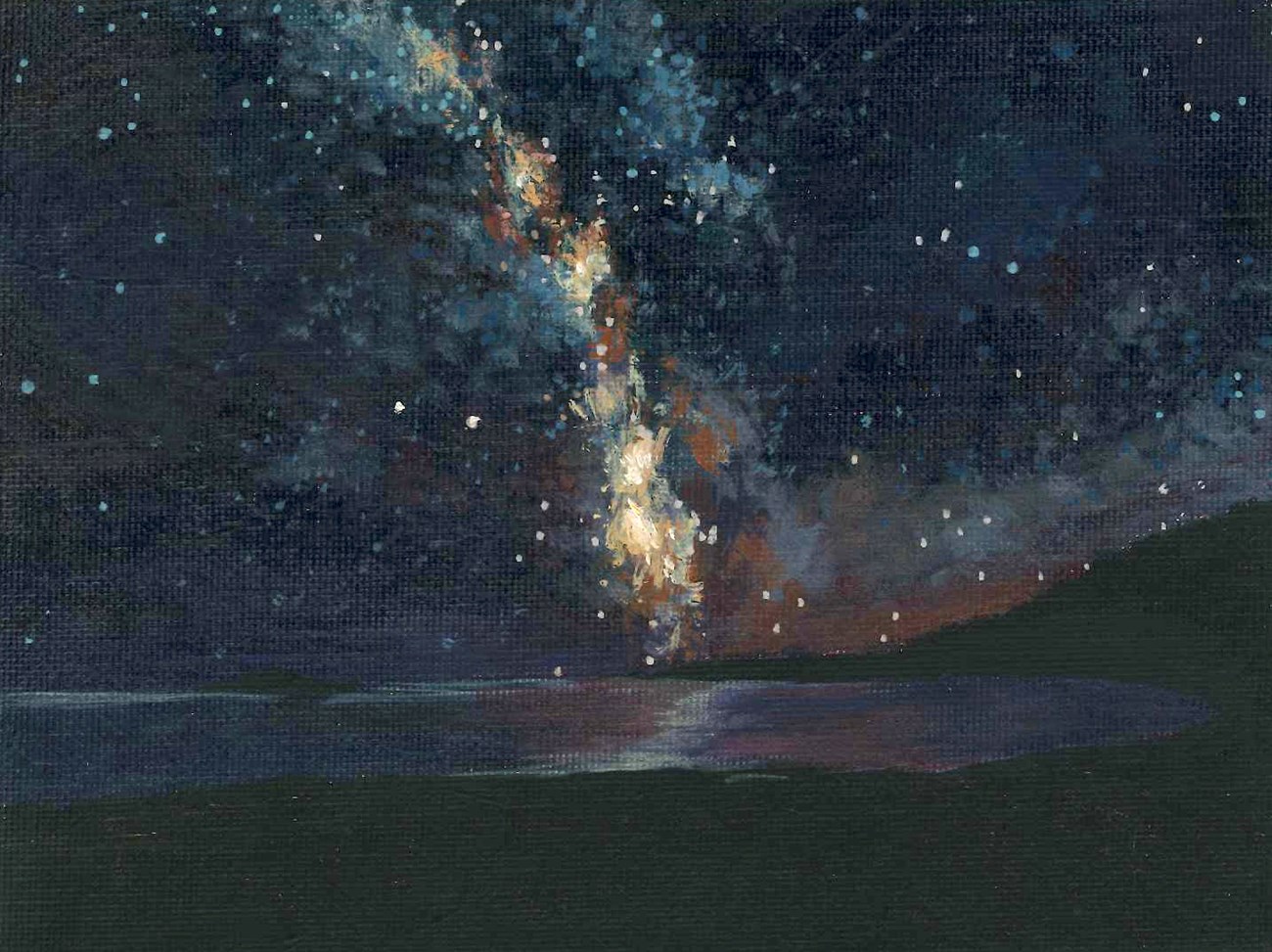This artistic painting, created on a textured canvas, vividly depicts a dramatic night sky over a serene landscape. The bulk of the image is enveloped in darkness, suggesting a deep night, with rich dark blue hues dominating the sky. Scattered throughout are white and bluish circles representing stars, adding a celestial charm. There are also intriguing bursts of rust, brown, and cream colors, resembling a nebula or celestial fire, creating an explosion of colors. Below the sky, a pitch-black landmass, indicative of nightfall, stretches across the bottom. In front of it lies a reflective body of water, tinged with dark blue and hints of white and red, likely mirroring the vibrant sky above. On the right-hand side, a faint, greenish hill or mountain can be seen, adding depth and contrast to the composition. This breathtaking nightscape not only captures the stillness of a night by the water but also the awe-inspiring beauty of cosmic phenomena.